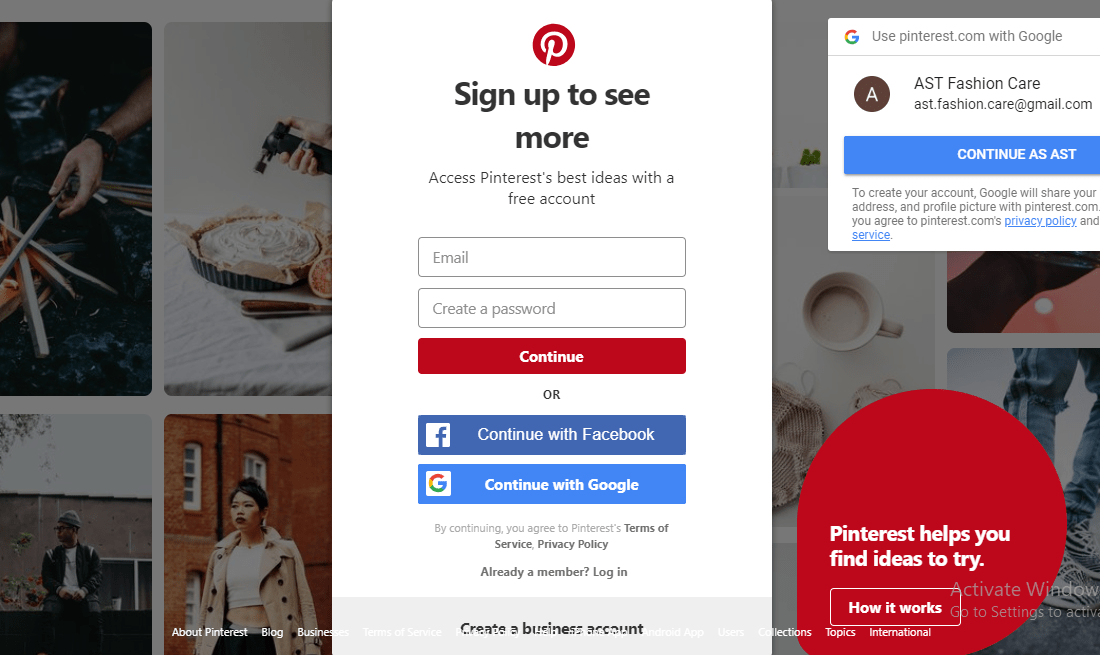This landscape-oriented photo captures the Pinterest sign-up or homepage, featuring a central white vertical box. At the top of this box, the recognizable red Pinterest logo—a white cursive "P" inside a red circle—stands out. Below, in black text, is the prompt: "Sign up to see more and access Pinterest's best ideas with a free account." The box provides fields for entering an email and password, accompanied by a prominent red "Continue" button with white text. Alternatively, users can log in with Facebook or Google, with their respective logos displayed in matching colors.

To the left, a vertical section showcases four pictures: one depicts a hand holding some sticks, another shows a person torching or baking a pie, the third features a man leaning against a wall, and the fourth displays a woman in a short shirt and long jacket standing beside a building.

On the right, another vertical section contains a white pop-up box inviting users to use Pinterest.com with Google. Below this prompt, an account option is shown with a brown circle and white "A" labeled "AST Fashion Care," along with a blue "Continue as AST" button. Beneath this, a red circle with white text reads, "Pinterest helps you find ideas to try."